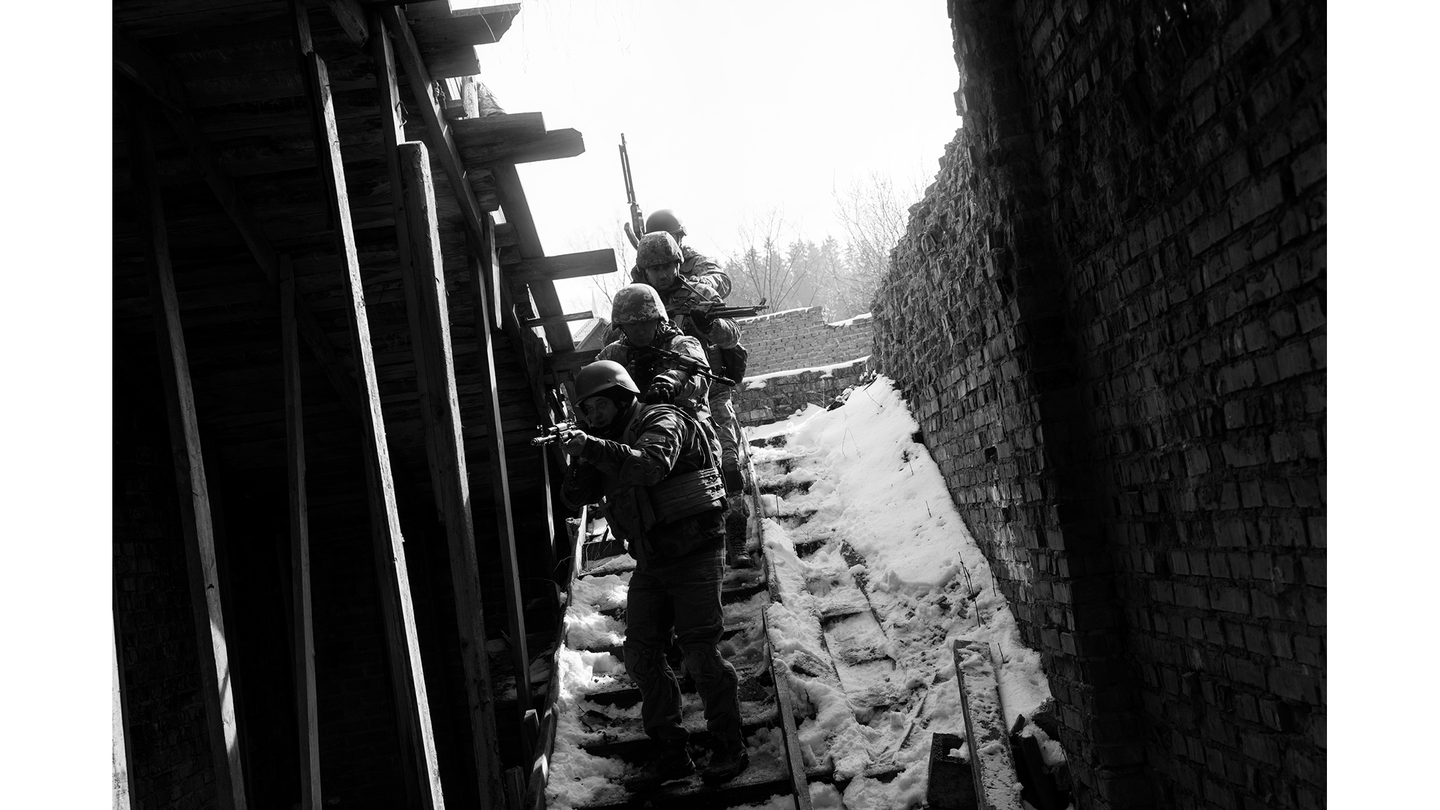This is a black-and-white wartime photograph capturing four armed soldiers descending a snow-covered wooden staircase. Each soldier is carrying a rifle, with some pointing forward and the rear soldier holding his rifle up in the air. To the right of the staircase is an exposed, weathered brick wall that adds to the historical atmosphere of the scene. To the left, the staircase is bordered by a wooden structure or barricade. In the background, an overcast sky and distant trees frame the stark winter setting, emphasizing the harsh and austere conditions.